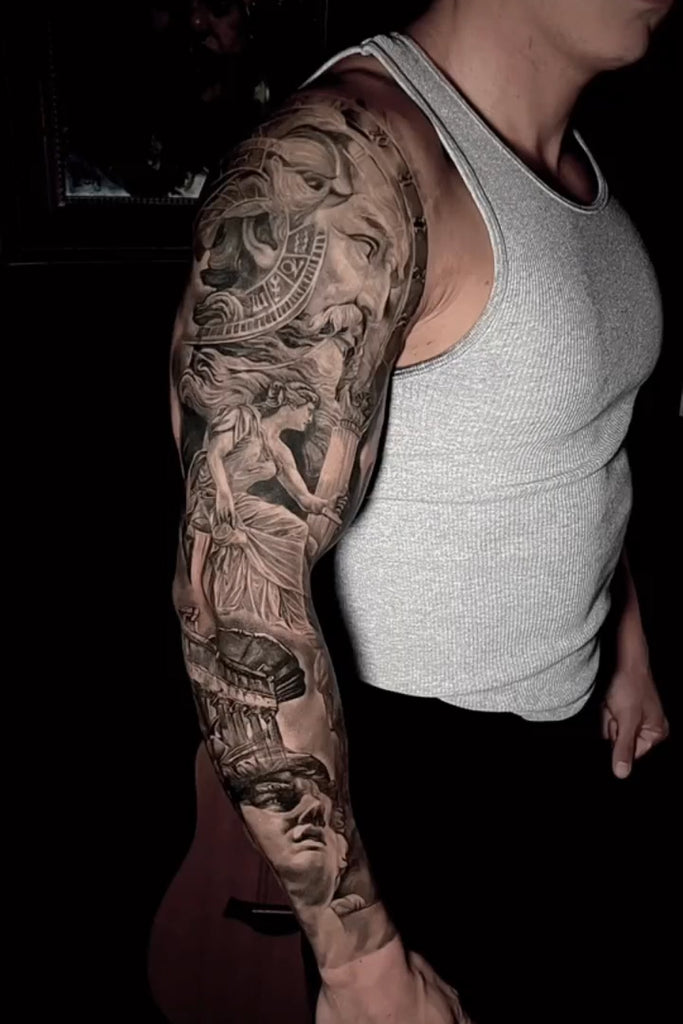This is a detailed photograph focusing on a person's right arm, which features an ornate and highly detailed black and white sleeve tattoo. The individual is wearing a grey tank top and standing with their body facing the right while their head is partially cropped out of the frame. The person is muscular, fair-skinned, and their fists are clenched down by their sides. The background is mostly dark, with an acoustic guitar leaning against the wall and a faint reflection of a man with a goatee in a window. Behind him, a black wall is visible.

The tattoo, depicted in a realistic classical style, showcases various Greco-Roman figures, including what appears to be Zeus and other gods. These figures are intricately designed, showing different emotions ranging from confusion to deep thought. The woman in the middle of the tattoo wears a flowing dress and seems confused, while the man at the bottom expresses disgust. The man at the top has sightless eyes, a thick mustache, and a receding hairline, appearing deeply contemplative. Surrounding these figures are numerous ornamental details, including symbols of the zodiac, sundial-like elements, and classical columns, all intricately blended together in a cohesive and visually striking design.